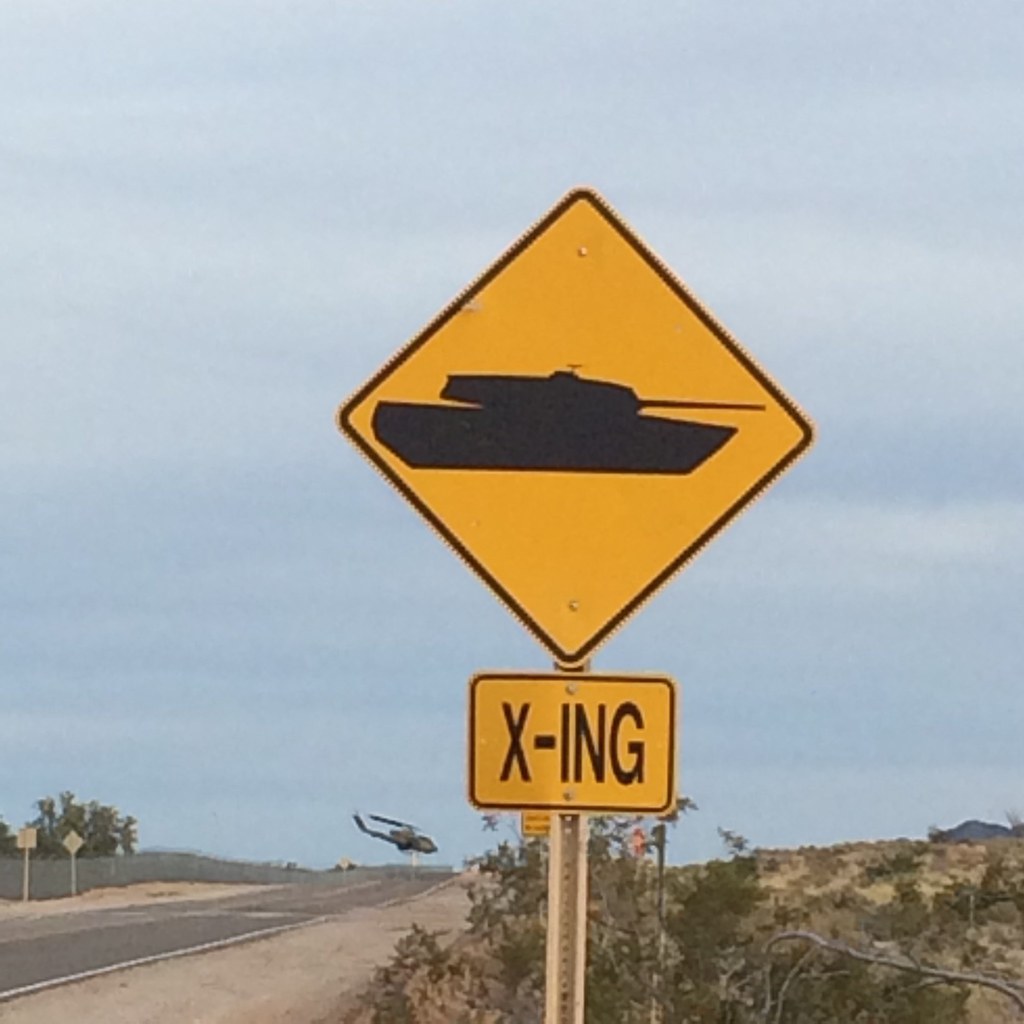Captured in the image is a rural road bordered by coarse gravel on both sides. A lengthy fence runs alongside the right side of the road, interspersed with trees and street signs. On the right side of the road, dried land dotted with sparse patches of green and brown stretches out under an expansive blue sky. In the distance, a large, dark-colored military helicopter prepares to land, its imposing bulk contrasting with the surroundings. Near the foreground, a notable street sign stands: a silver pole holds up a large yellow sign, bordered in black, featuring the silhouette of a tank. Beneath it, a smaller sign reads "X-ing" in bold black letters on a yellow background.